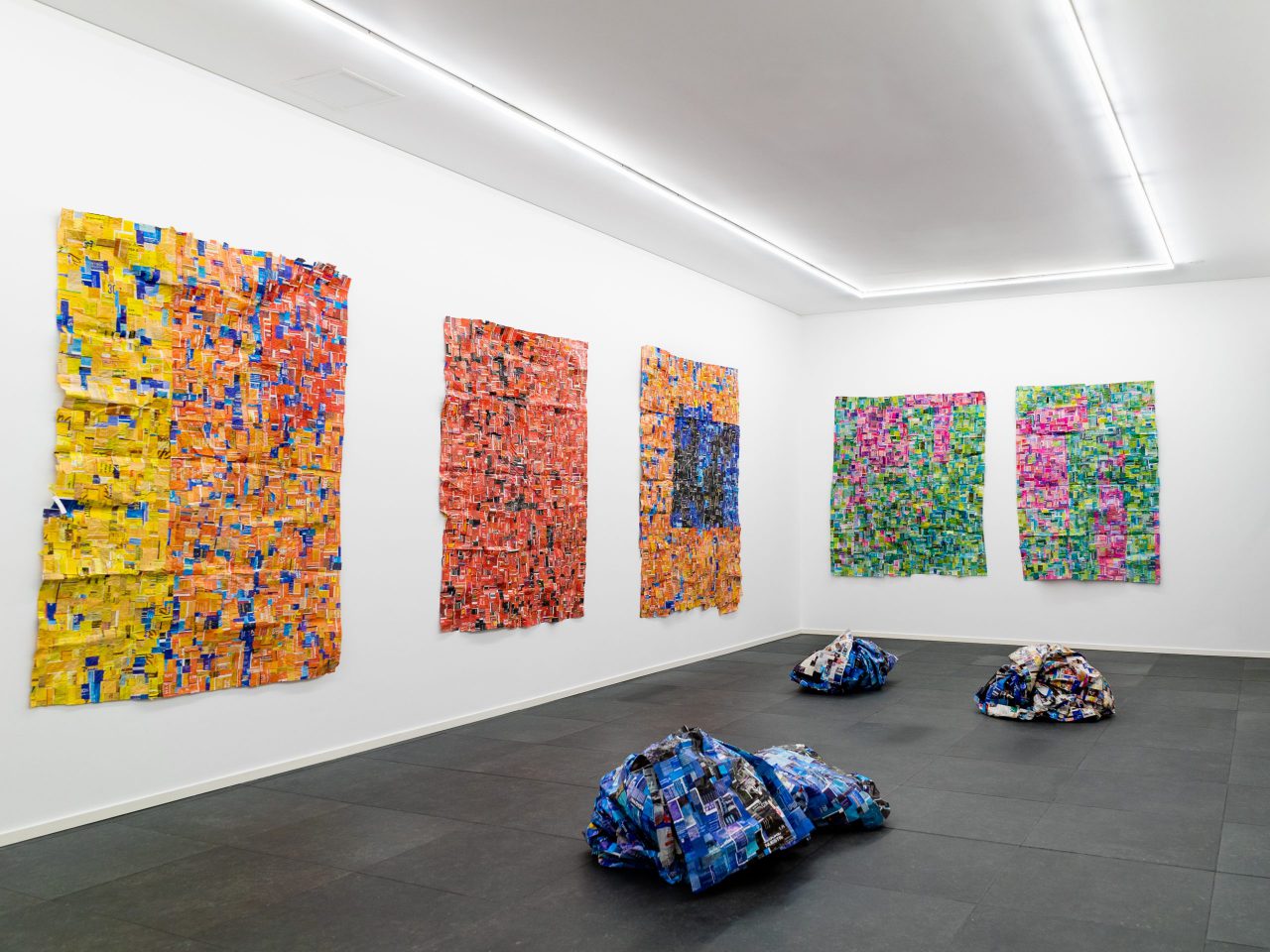The image likely represents a hyper-realistic digital art gallery with a sleek modern design, featuring white walls, a silver or gray ceiling with a rectangular array of bright lights, and a black floor. On the left wall, there are three evenly spaced paintings constructed from labels of the same hue, creating a cohesive visual theme. These labels seem to mimic the appearance of pixel art with each painting exhibiting a distinct color theme—predominantly orange, yellow, and red hues. On the back wall, there are two more paintings, also resembling pixel compositions but utilizing green and pink shades to create plant and floral imagery. 

Additionally, the floor displays three three-dimensional objects that appear to be piles of crushed metal, creatively wrapped in blue and white materials, echoing the pixel aesthetic with their textured, wrinkled surfaces. The front-most object is predominantly blue, while the two behind it are respectively blue and a mix of silver and gold, offering a striking contrast against the smooth, black floor.